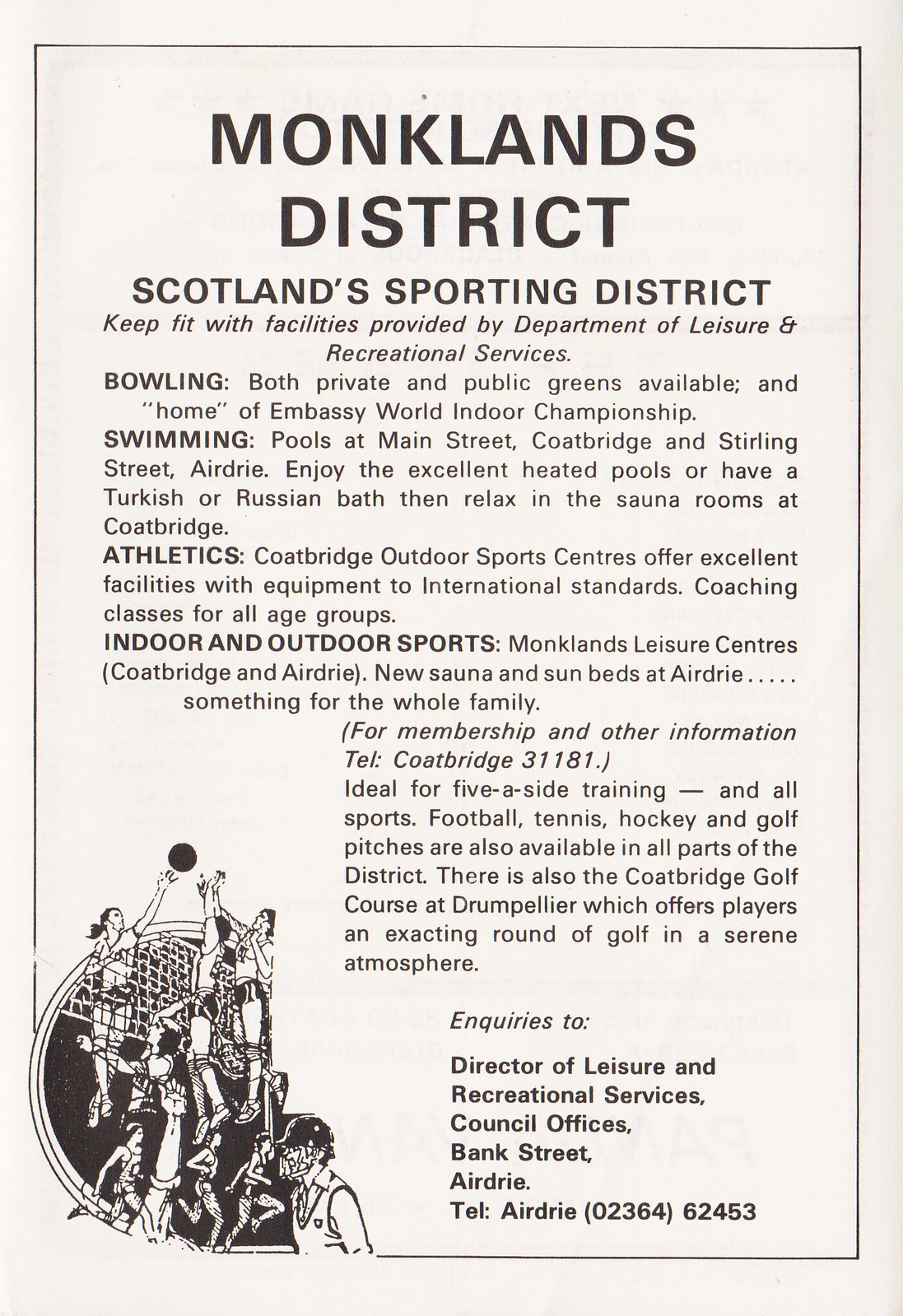The image is a portrait-sized poster with a solid tannish white background bordered by a thin black line. The headline, "Monklands District, Scotland's sporting district," is prominently displayed at the top in all caps, followed by a line encouraging fitness through facilities provided by the Department of Leisure and Recreational Services. The text is predominantly black, detailing various activities such as bowling, swimming, and athletics, with specific highlights on facilities like private and public bowling greens and swimming pools located at Main Street, Coatbridge, and Stirling Street, Airdrie. In the bottom left corner, there's a hand-drawn, cartoon-like graphic depicting people running, playing volleyball, and jumping, along with a coach or referee wearing a helmet. The poster, entirely in black and white, concludes with additional information including a phone number and address for further inquiries.